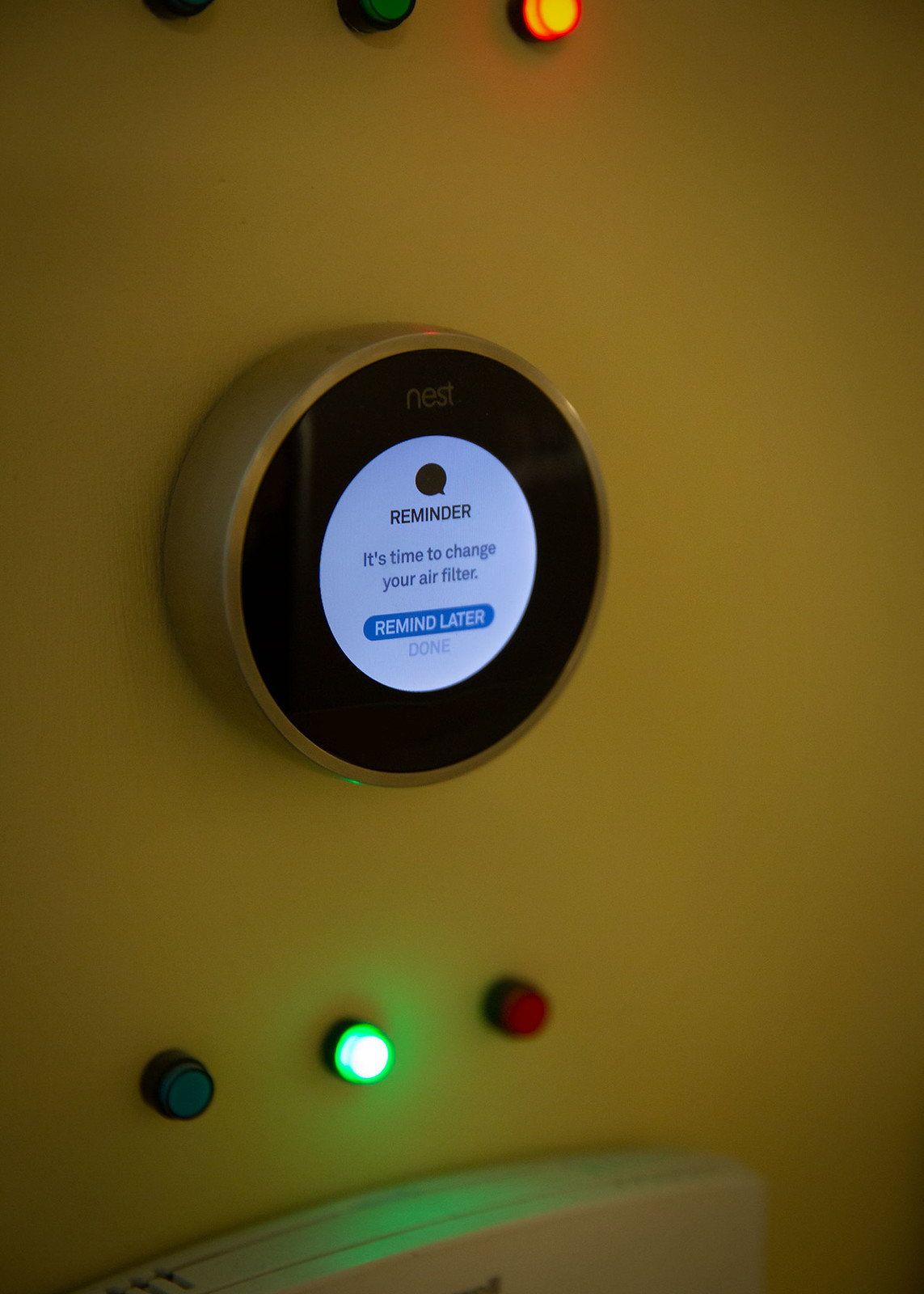The image depicts a smart thermostat, specifically a Nest model, mounted on an off-white, slightly yellowed wall. The thermostat is designed with a sleek silver, chrome-like finish, and prominently displays a black circular interface at its center. The middle of the interface features a bright blue background with a message symbol. The message displayed reads, "Reminder: It's time to change your air filter," in light blue text.

Above the thermostat, there is a row of three indicator lights. The first indicator is green, partially visible from the left edge. The middle indicator is also green and fully lit. The third indicator is red and lit up. Below the thermostat interface, another set of three smaller lights is present. The first is green, the middle light is also green and lit up, and the last light is red.

In addition, at the bottom of the device, there is a white mark, suggesting some wear or a possible imperfection. The overall image captures a functional and well-used home appliance, highlighting its digital reminder features and sophisticated design.